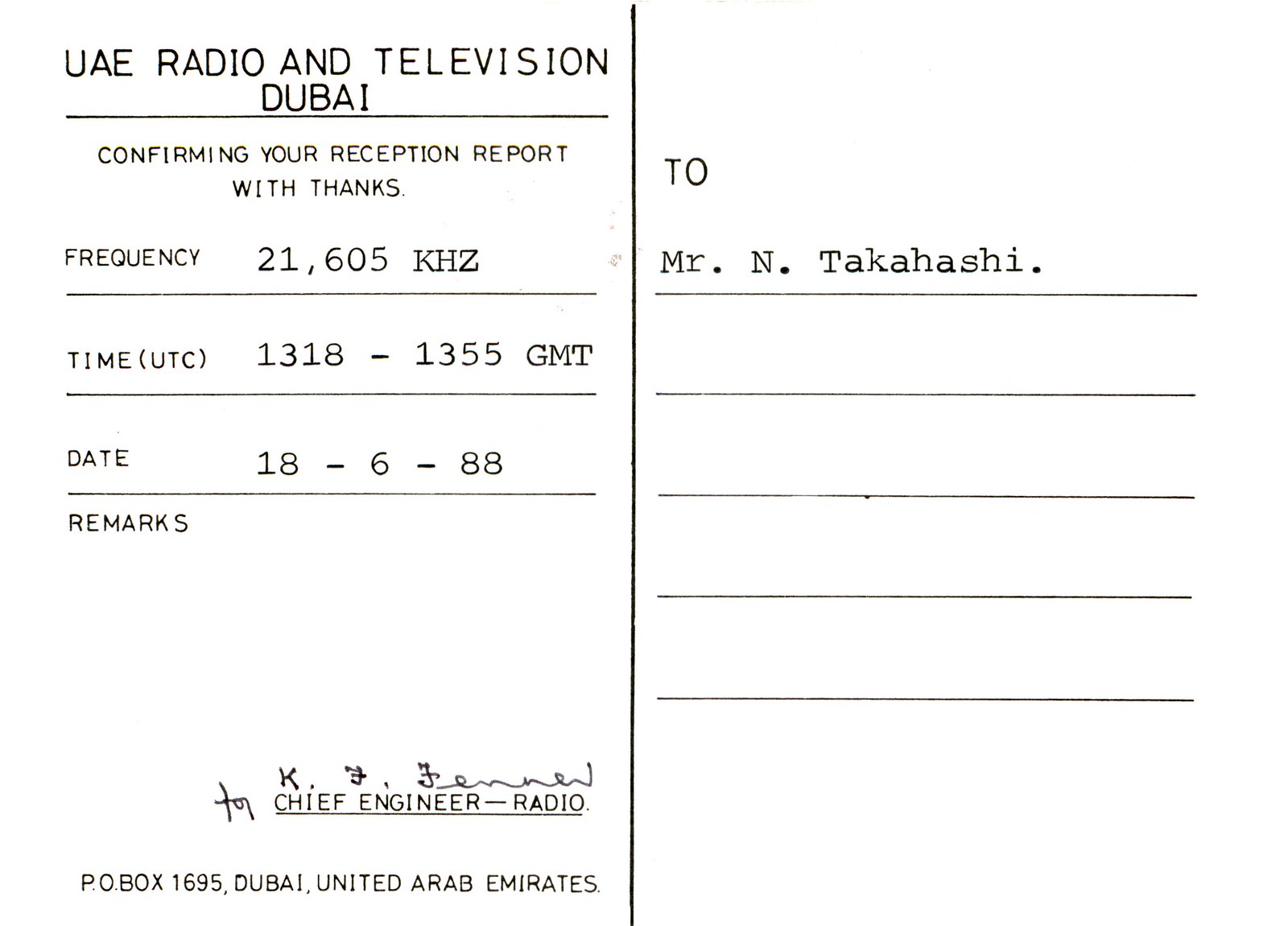**Detailed Caption:**

The image depicts an official receipt confirming the reception report. The text, printed in black on a white background, reads "UAE, United Arab Emirates, Radio and Television, Dubai." The receipt acknowledges the reception with gratitude, providing specific details such as frequency, time, and date. The recipient of this confirmation is Mr. N. Takashi. The document follows a left-to-right layout typical of receipt formatting, including a time stamp and date. It bears the signature of the Chief Engineer of Radio and lists the address as PO Box in Dubai, United Arab Emirates.